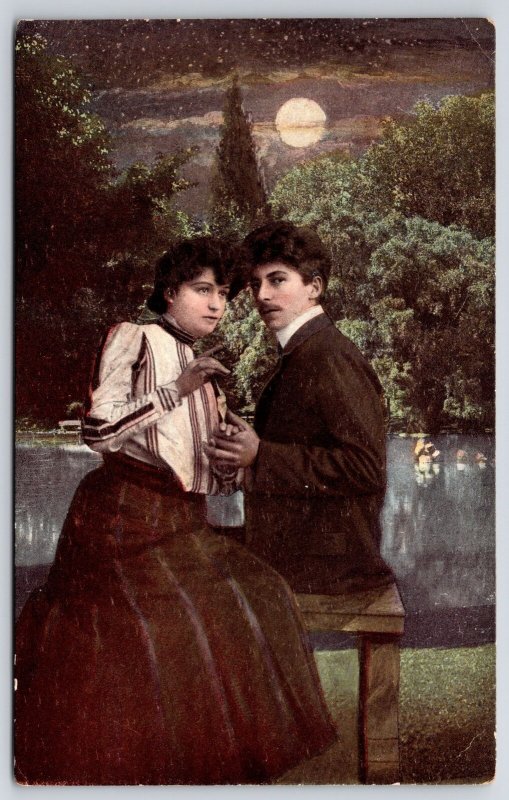The image depicts a seemingly vintage scene, perhaps from the 1920s, featuring a man and woman seated on a wooden bench by a serene body of water. The duo appears serious and somewhat suspicious, with the woman pointing at something while they both gaze in the same direction. She dons a black skirt and a white blouse adorned with stripes or brown trim, complemented by her black hair styled in a manner characteristic of the era. The man, in a suit with a white collar and sporting a mustache, is turned to the side, revealing the left profile of his face. They hold hands, creating a sense of connection. Behind them, the landscape includes lush green trees and bushes, leading to a tranquil lake. The scene is bathed in the ethereal glow of a full moon, surrounded by stars and clouds, indicating it's nighttime. The background also features a concrete ledge adding to the picturesque outdoor setting that resembles a classic European locale such as Paris.